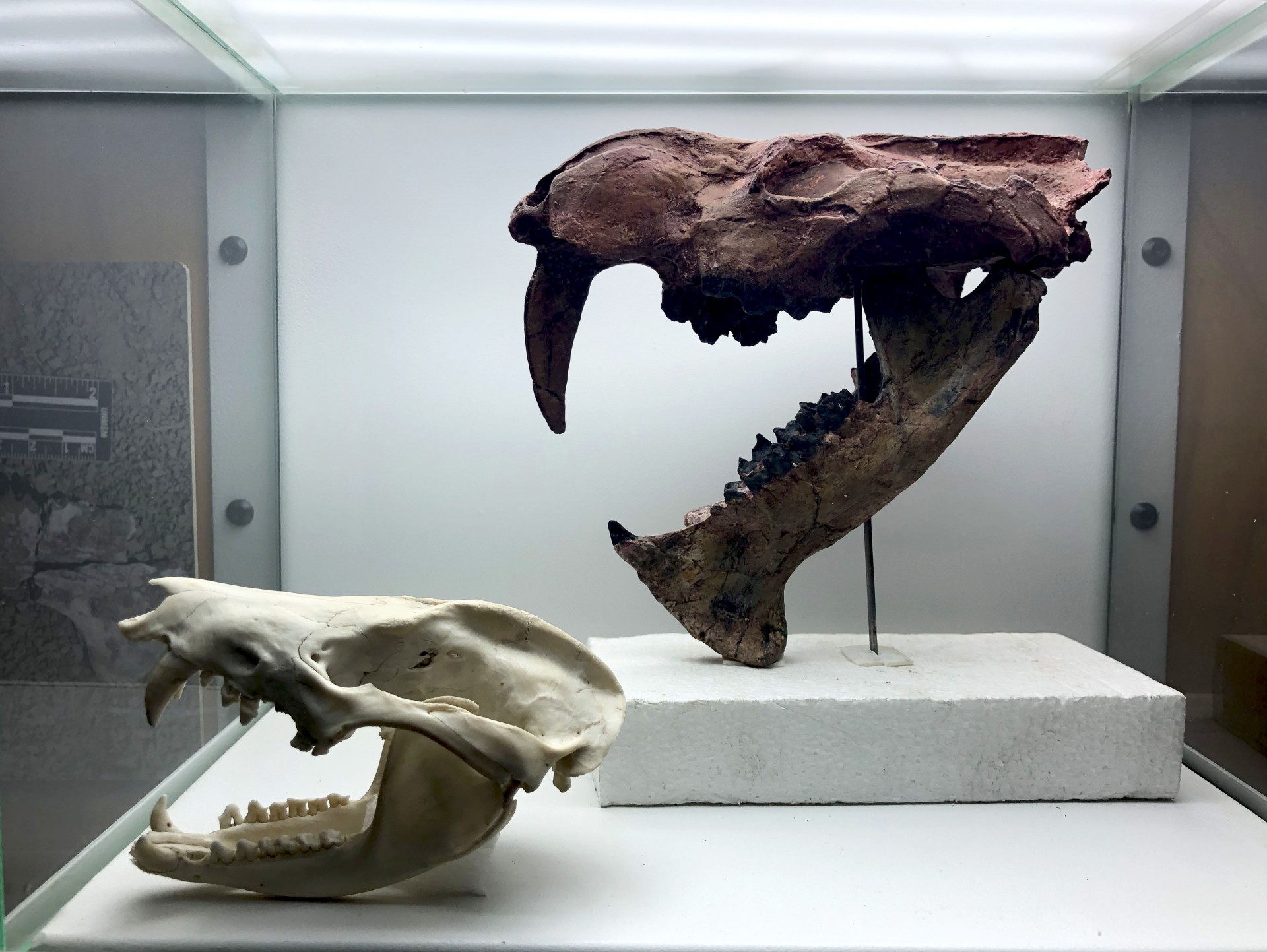The image depicts a detailed display within a museum exhibit. Encased in a rectangular glass box with a white back panel, the exhibit showcases two prominent animal skulls, possibly of dinosaur or saber-toothed tiger origin. The larger skull, brown in color with distinct eye sockets, features a notably long, sharp tooth extending from the top jaw and various smaller teeth along the upper and lower jaws. This skull is supported by a thin metal dowel mounted on a white, rectangular stone block. The skull's mouth is propped open, displaying its intimidating dentition.

In front of and slightly to the left of the larger skull lies a smaller, white skull, seemingly a sculpted model. This skull also has a sizable fang protruding from the top and an array of teeth on the bottom jaw. Noticeably, there is a smooth, non-broken section in the skull's back, suggesting a missing piece of the structure. Both skulls are enclosed within the glass case, providing a clear view of their anatomical features and differences.